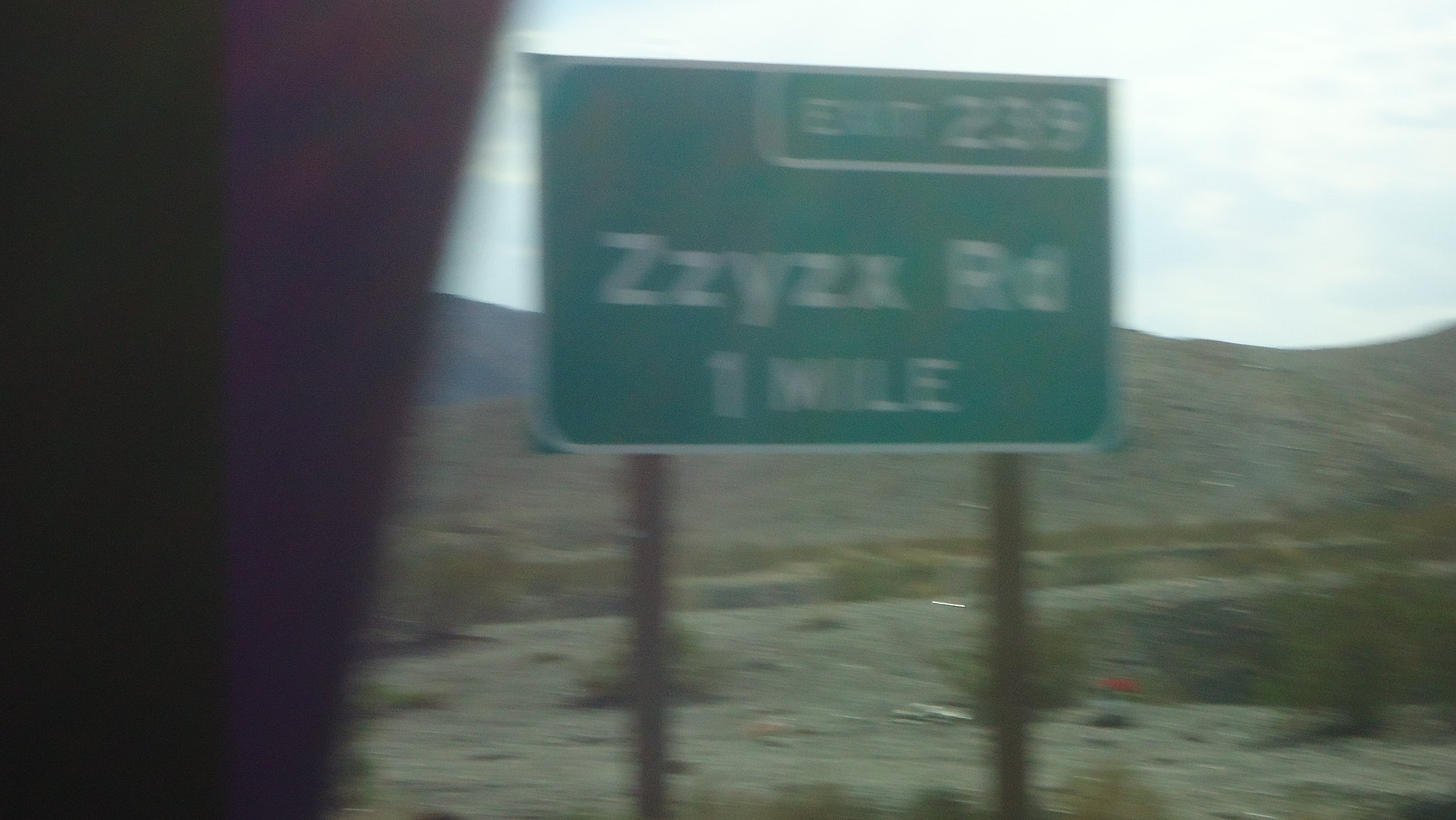In this color photograph taken from inside a moving car, we see a large green freeway exit sign that reads "ZZYZX Road, 1 Mile," with "Exit 239" prominently displayed at the top. The image captures the motion blur typical of a moving vehicle, with part of the car's interior and frame visible along the left edge. The background showcases an arid, mountainous desert landscape under a clear blue sky. The sign is supported by two steel poles, and the foreground includes some dirt and sparse grass along the roadside. Despite the blur, the green sign with its white trim and their respective details stand out against the stark scenery.